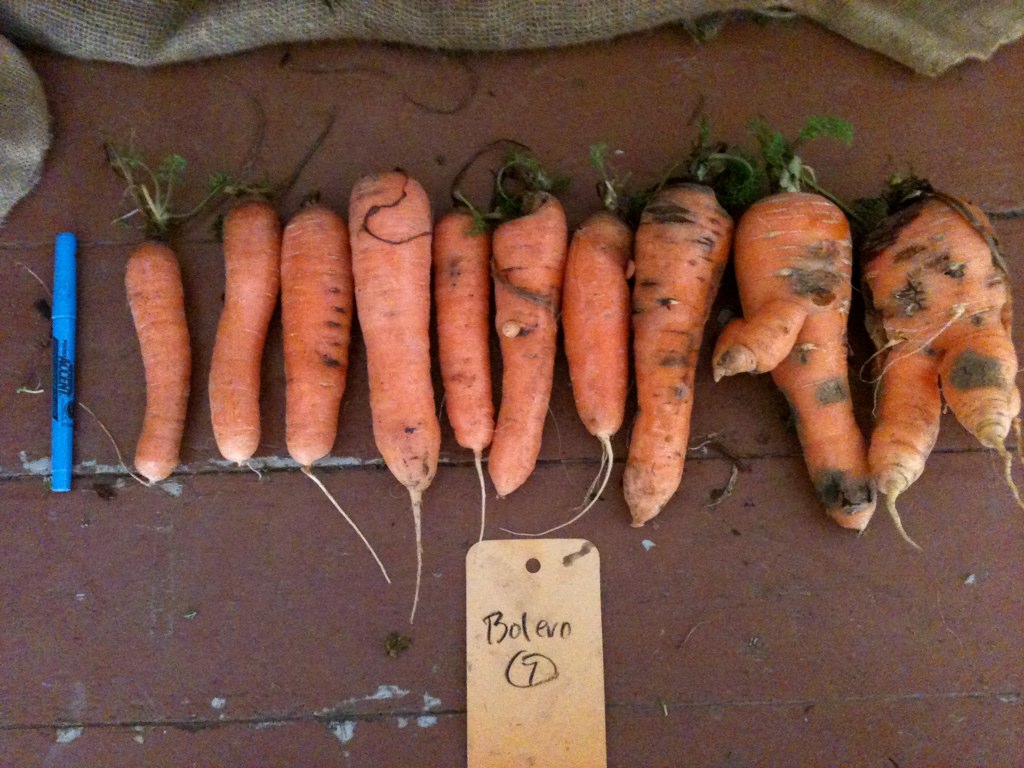This image displays a row of approximately ten organically grown carrots placed on a reddish-brown cement surface. These carrots exhibit considerable variation in size, shape, and texture. As you move from left to right, the carrots become increasingly mottled, damaged, and misshapen with noticeable brown spots and outgrowths. Some retain their green leafy tops, indicating they are fresh from the ground and not store-bought. An off-white tag below the carrots reads "Bolero 9," with the number circled. For size reference, a blue magic marker with its cap on is positioned to the left of the carrots. The overall scene is captured from a top-down perspective, giving a clear view of the irregular and earthy nature of the vegetables.